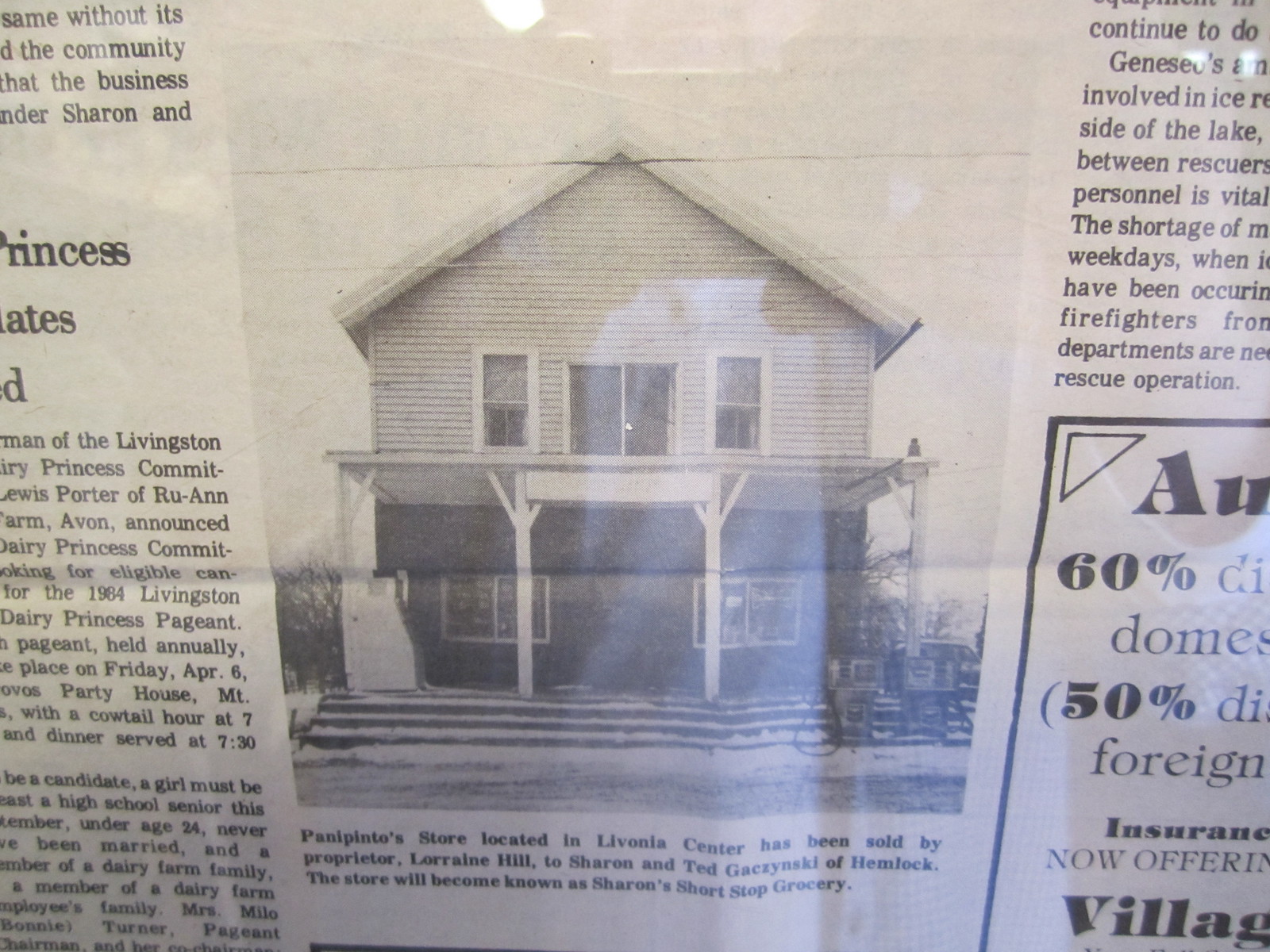This is a detailed photograph of a black and white newspaper clipping, capturing a notable transformation of a property in Livonia Center. The focal point is a two-story wooden house with vinyl or laminate siding, flaunting distinctive architectural elements: two upper-story windows, two large lower-story windows, and a centrally located door accessed via a porch and stairs. Beneath this house image, the caption reads: "Panepinto's store located in Livonia Center has been sold by proprietor Lorraine Hill to Sharon and Ted Kaczynski of Hemlock. The store will become known as Sharon's Short Stop Grocery." The newspaper clipping is placed behind a glass casing, causing a reflection in the photograph. Surrounding the image are multiple paragraphs and articles, with glimpses of words like "firefighters" and "60% and 50%" on the right, and "princess," "Sharon," "Livingston," and "Porter of Ruan" on the left, indicating partial yet diverse content. An advertisement is also visible in this detailed snapshot of the newspaper page.